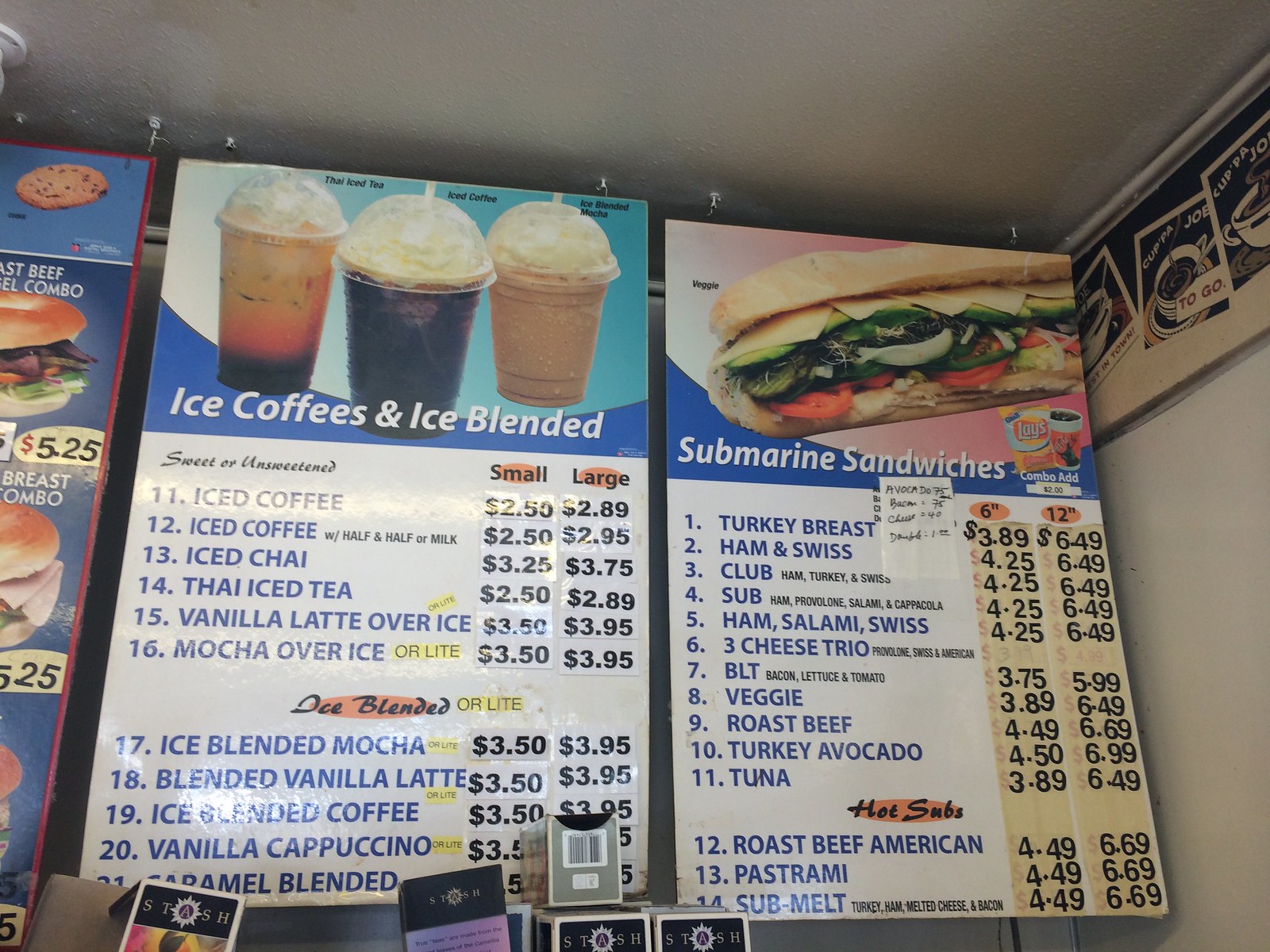This image captures the menu of a cozy tea and sandwich cafe, showcasing a variety of refreshing beverages and delicious submarine sandwiches. The menu is divided into several sections: Iced Coffees, Iced Blended Drinks, and Submarine Sandwiches. 

In the Iced Coffees section, patrons can choose from small and large sizes, with options such as:
- Iced Coffee ($2.50 for small, $2.89 for large)
- Iced Coffee with Half and Half or Milk
- Iced Chai 
- Thai Iced Tea ($2.50 for small, $2.89 for large)
- Vanilla Latte over Ice
- Mocha over Ice ($3.50 for small, $3.95 for large)

Moving to the Iced Blended section, the menu features sweetened and blended delights:
- Iced Blended Mocha
- Iced Blended Vanilla Latte
- Iced Blended Coffee
- Iced Vanilla Cappuccino
- Caramel Blended Drinks

The range of Submarine Sandwiches includes options for every taste preference, available in 6-inch and 12-inch sizes:
- Turkey Breast ($3.89 for 6-inch, $6.49 for 12-inch)
- Ham and Swiss Club
- Ham, Salami, Swiss
- Three Cheese Trio
- BLT
- Veggie
- Roast Beef
- Turkey Avocado
- Tuna
- Roast Beef American
- Pastrami ($4.49 for 6-inch, $6.69 for 12-inch)
- Sub Melt

Additionally, the image includes visuals of the delectable subs and topped iced teas, many adorned with generous dollops of whipped cream. On the left side, there are other food items and various utensils or supplies neatly stacked at the bottom. The detailed pricing and the variety of around 25 different items make this menu both appealing and pocket-friendly.